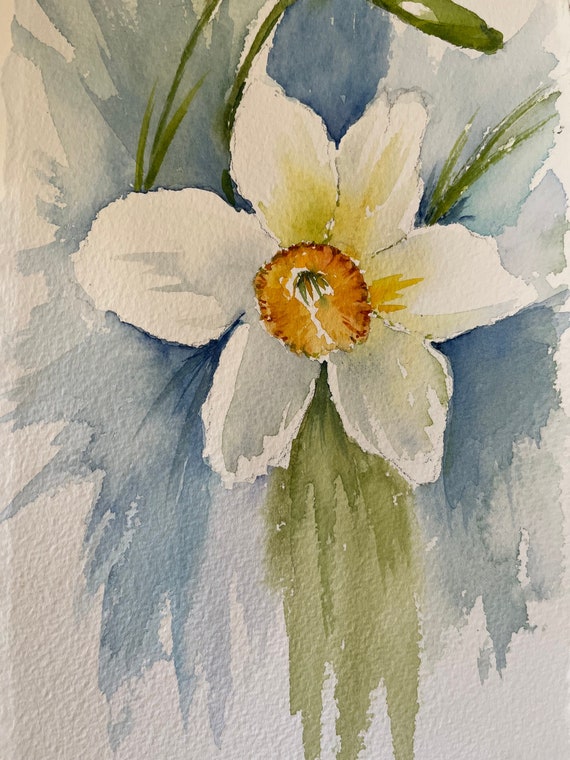This is a vertically oriented watercolor painting of a single white daffodil. The daffodil, which dominates about a third of the composition, is artfully rendered with white petals and a vibrant orange center, accented by yellow reflections. The flower's cup features darker green stamens, adding depth to its intricate details. Surrounding the daffodil is a blend of green foliage, likely depicting stems and leaves, and some watercolor washes in light blues and grayish blues that evoke a serene sky. Parts of the background also include areas left unpainted, exposing the white of the canvas and enhancing the airy feel of the scene. Above the daffodil, some clearer green lines suggest additional leaves or a budding flower, adding a touch of natural complexity to the elegant simplicity of the single bloom.